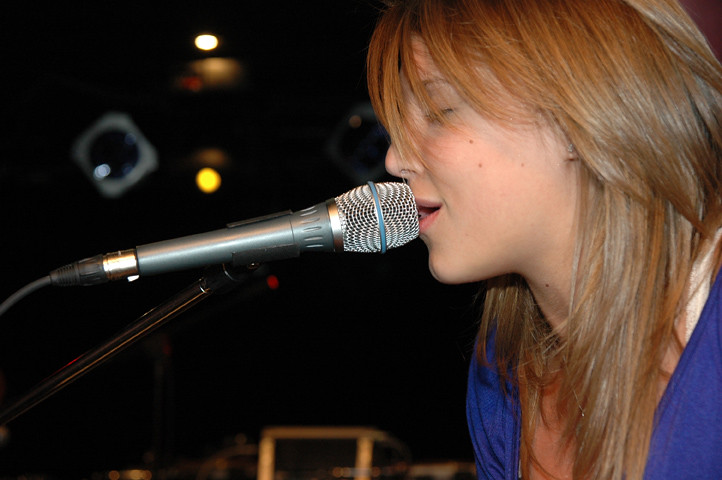In the close-up image, a woman with light brown-to-dark blonde hair sings passionately. Her hair, cut with longer bangs, partially obscures her closed eyes and almost covers her nose, of which only the very bottom peeks out. Her mouth is pressed right up against a silver microphone adorned with a blue band, emphasizing her engagement in the song. The woman wears a royal blue V-neck shirt, slightly cut off at the bottom of the image to show parts of her chest and the edges of a white tank top beneath. Her face, turned to the left, reveals light skin with moles on her cheek and neck, and she dons a clear stone earring along with a silver necklace. The background features a blurry, dark setting speckled with yellow lights, suggesting she is performing on a stage.